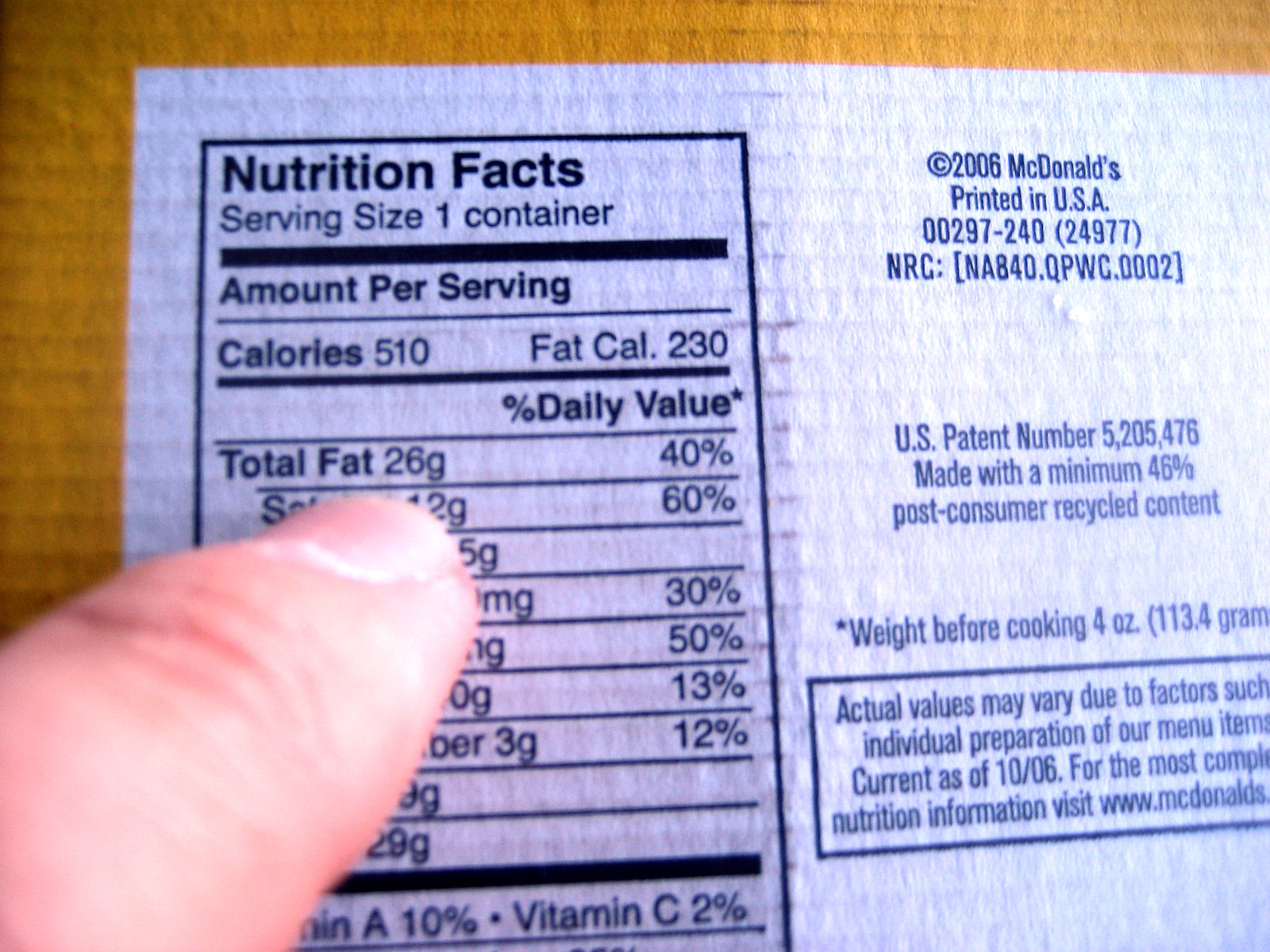A detailed close-up photograph captures the backside of a McDonald's cardboard box, focusing on its nutritional information. A pudgy Caucasian index finger, appearing slightly rough and worn, prominently points toward the "Total Fat" section of the nutritional facts. The printed details reveal that the "Serving Size" is one container, containing 510 calories, with 230 of those calories derived from fat. The "Total Fat" content is specified as 26 grams, which constitutes 40% of the daily recommended value. The black ink nutritional data is stamped clearly on a white graphic printed on the box, while the rest of the information is obscured by the pointing finger.